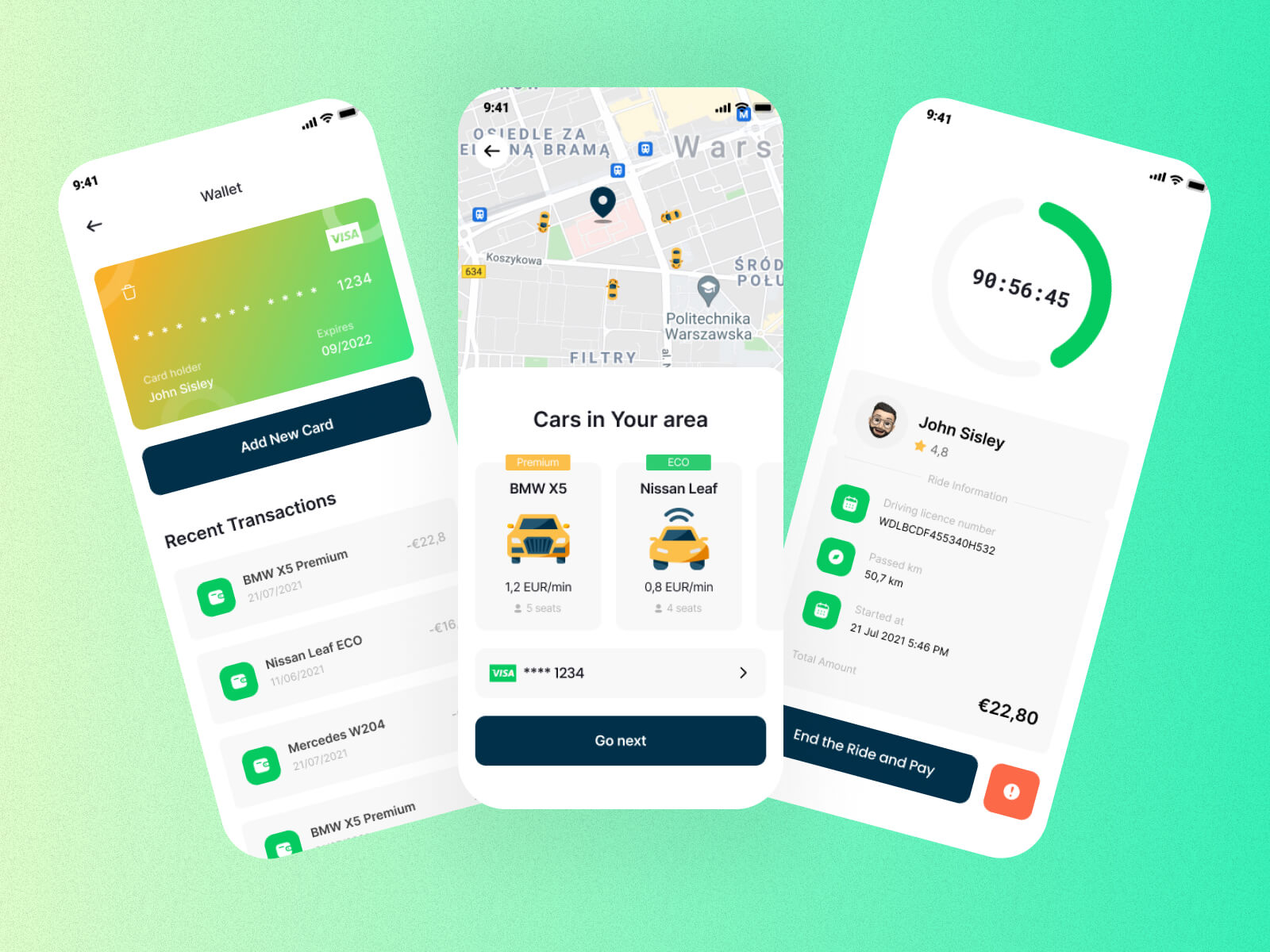The image depicts a comprehensive advertisement for a ride-share application, showcasing three crucial screenshots that highlight the app's key features.

The first screenshot presents the "Wallet" section of the app, displaying a digital credit card interface. It includes an "Add New Card" option and a list of recent transactions. Notably, transactions shown include purchases like "BMW X5 Premium," "Nissan Leaf Eco," and "Mercedes W204."

The second screenshot focuses on the ride-sharing service's map feature. It displays a map pinpointing available cars in the area, including details such as car models like "BMW X5" and "Nissan Leaf." Users' payment information involving VISA can be seen at the bottom, along with a "Go Next" button to proceed.

The third screenshot highlights the ride’s progress. It features a circular time display, an icon of the driver John Sisley who has a 4.8-star rating, and details about the driving license, distance covered (KM), starting date, and the estimated cost of the ride. A button labeled "End Ride and Pay" is available for concluding the trip.

The background of the app consists of a gradient transitioning from light green to a mildly darker green, providing a soothing and modern interface design.